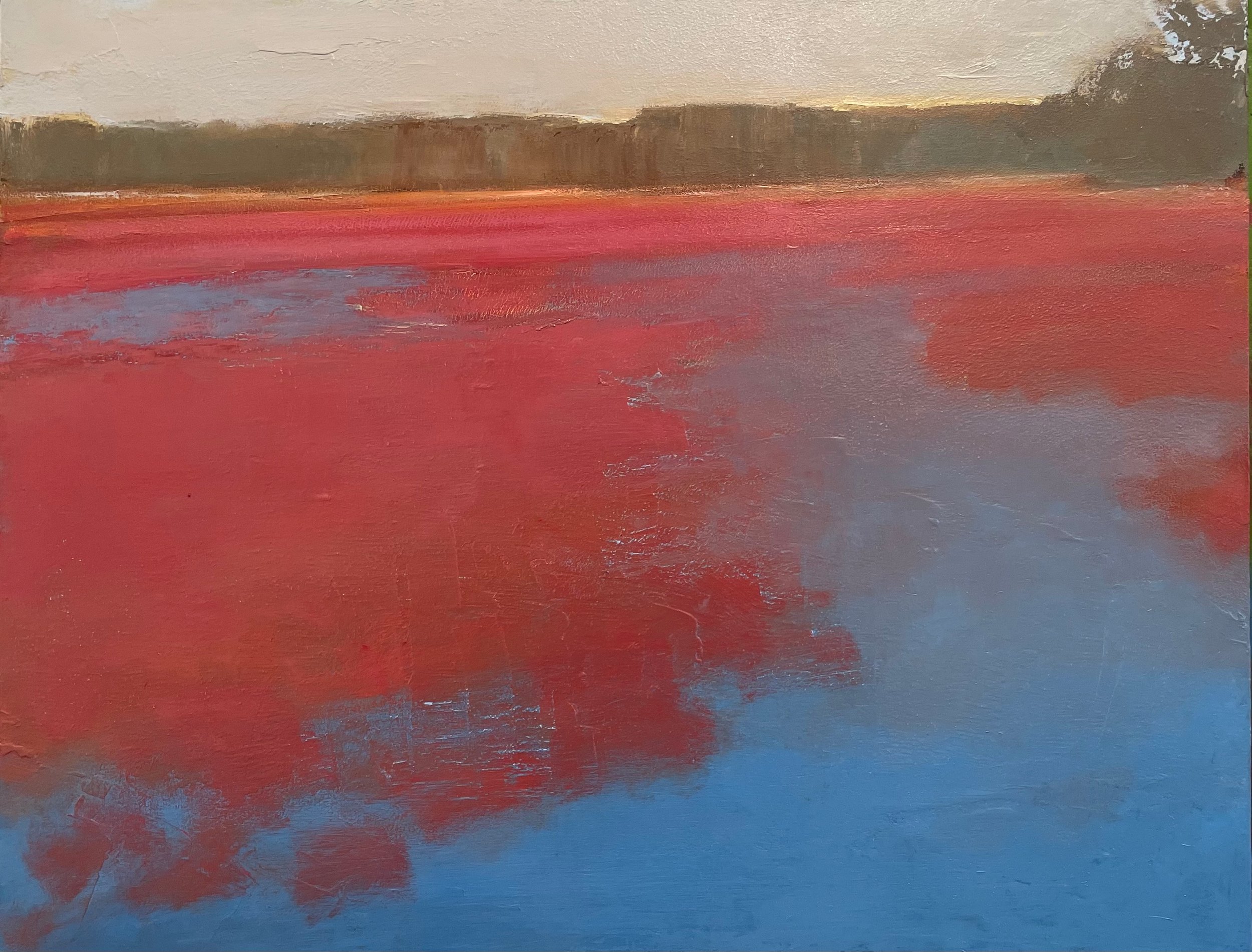This abstract watercolor painting portrays a vividly striking lake where the water is predominantly red, intertwined with patches of blue, giving it an unsettling and somewhat eerie appearance, reminiscent of blood or red algae. Beyond the lake, a vast brown cliffside stretches across the background, suggesting a formidable mountain range. The sky above this surreal landscape presents a gradient of colors, with a cream hue suggesting either the early moments of dawn or the final glow of dusk, interspersed with grey clouds. To the upper left and right corners, splotchy representations of tree branches or bushes overhang the water, adding to the layered depth of the scene. The overall style employs a sponge or spackle technique, enhancing the abstract and textured feel of the composition.